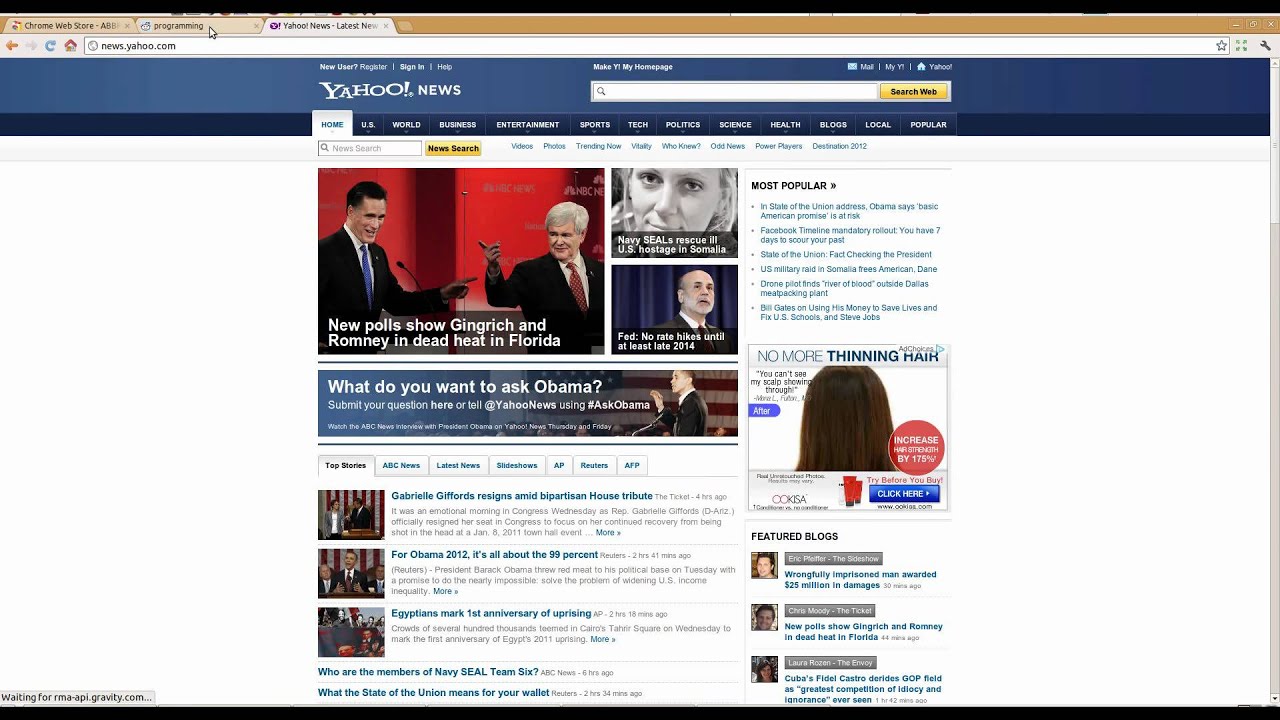The image depicts a computer screen showcasing multiple browser tabs and a Yahoo News webpage. At the top of the browser, there are three visible tabs. The first tab is for the Chrome Web Store, the second contains a webpage related to programming, and the third, highlighted tab is for Yahoo News. The URL in the search bar reads "news.yahoo.com," and the browser interface includes icons for back, forward, refresh, and home functions.

On the Yahoo News homepage, various sections are prominently displayed including Home, U.S., World, Business, Entertainment, Sports, Tech, Politics, Science, Health, Blogs, Local, and Popular. The top headline reads, "New Poll Shows Gingrich and Romney in Dead Heat in Florida," accompanied by an image of two men in suits, one wearing a red tie and the other a blue tie. 

Another headline states, "Navy SEALs Rescue Ill U.S. Hostage in Somalia," alongside a photograph of a woman. A third headline reads, "Fed: No Rate Hikes Until At Least 2014," with an image of a man in a suit.

The webpage also features a "Most Popular" section with various clickable blue headlines, suggesting popular news articles. An advertisement displaying "No More Thinning Hair" shows an image of brown hair from the back. Additionally, there is a "Featured Blogs" section with numerous blue clickable links, and a collection of top stories, giving the page the appearance of a typical news website.